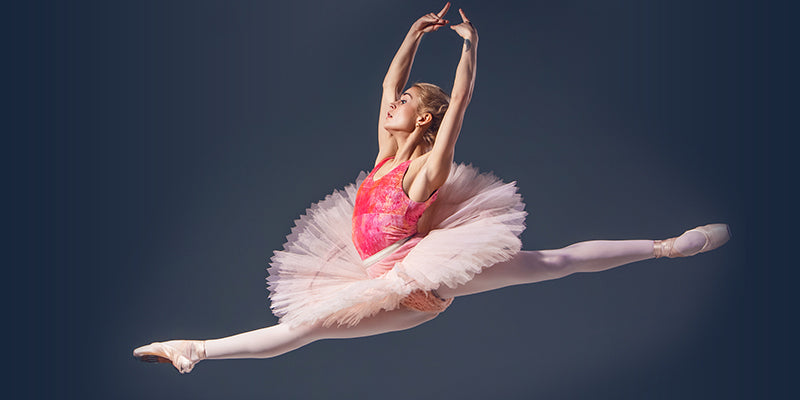The image portrays a blonde ballerina with short hair, gracefully suspended in mid-air during a split jump. Her legs extend dynamically, one stretched behind her and the other in front, showcasing her incredible flexibility. She is adorned in a light pink tutu with a ruffled, circular white skirt that flares out around her, paired with light pink leotards and pink ballet shoes. Her top is distinct with a tie-dye pattern of pink, orange, and red. Her arms are elegantly raised above her head, hands cupped together, emphasizing her poised form. Notably, a tattoo adorns her left arm near her hand. The backdrop of the image is a solid dark blue, contrasting sharply with her attire, and she's highlighted by stark lighting, emphasizing her presence against the background of the rectangular, horizontally oriented photo.